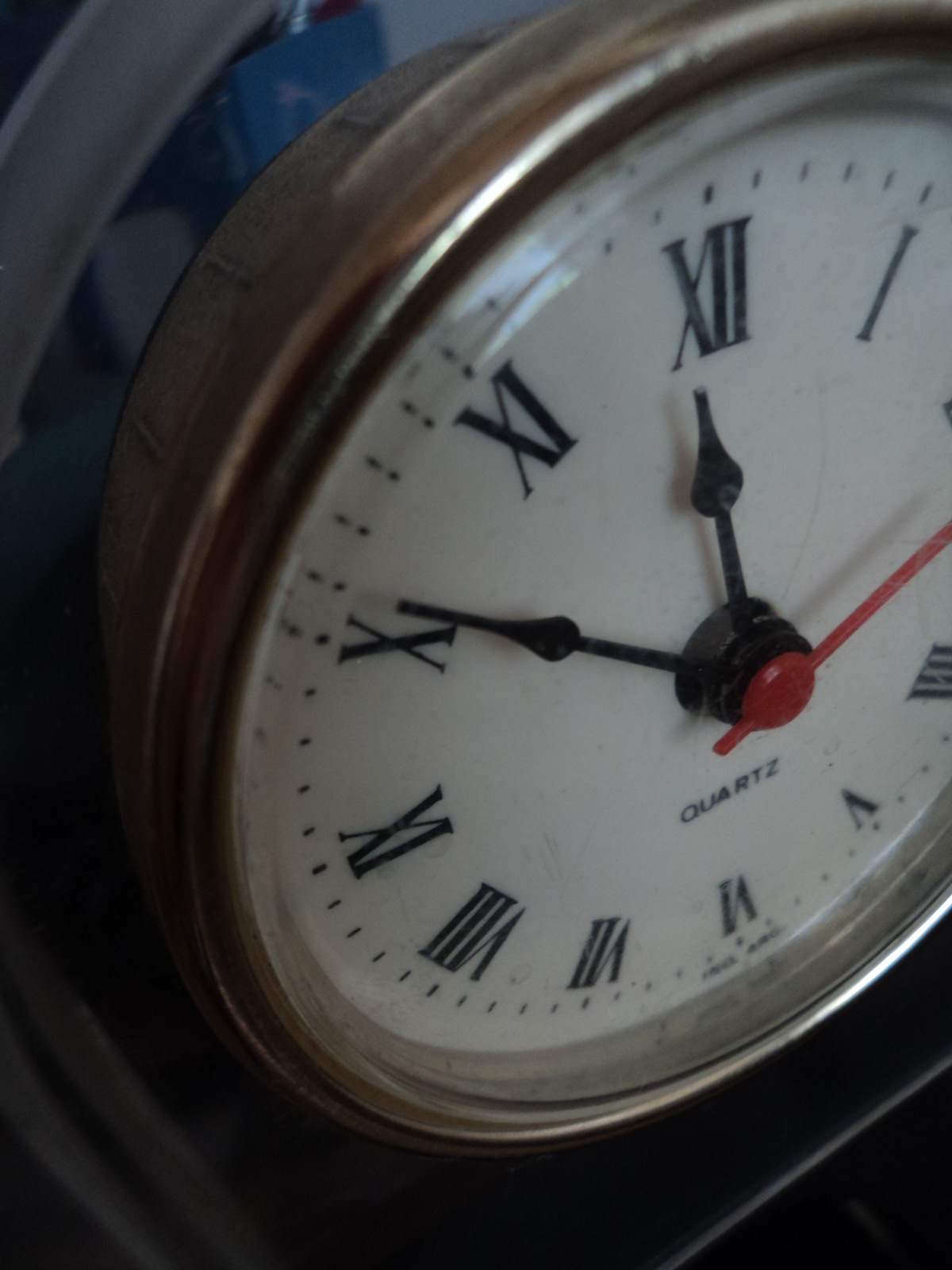This close-up image captures an intricately detailed clock face with a brass exterior and a white face adorned with black Roman numerals. The Roman numerals are displayed unconventionally, with some numbers oriented upside down, such as an inverted "V" for 5 and an upside-down "VI" for 6. The time indicated on the clock is 11:51, or 9 minutes to 12. The clock hands are black with teardrop-shaped ends, and there's a distinctive red second hand. The clock, which is predominantly featured in the image, bears the label "quartz" denoting its mechanism. There is a hint of blue in the top right corner of the background, possibly indicating an object like a book. The scene is somewhat dark and shadowy, with the clock taking up most of the frame.